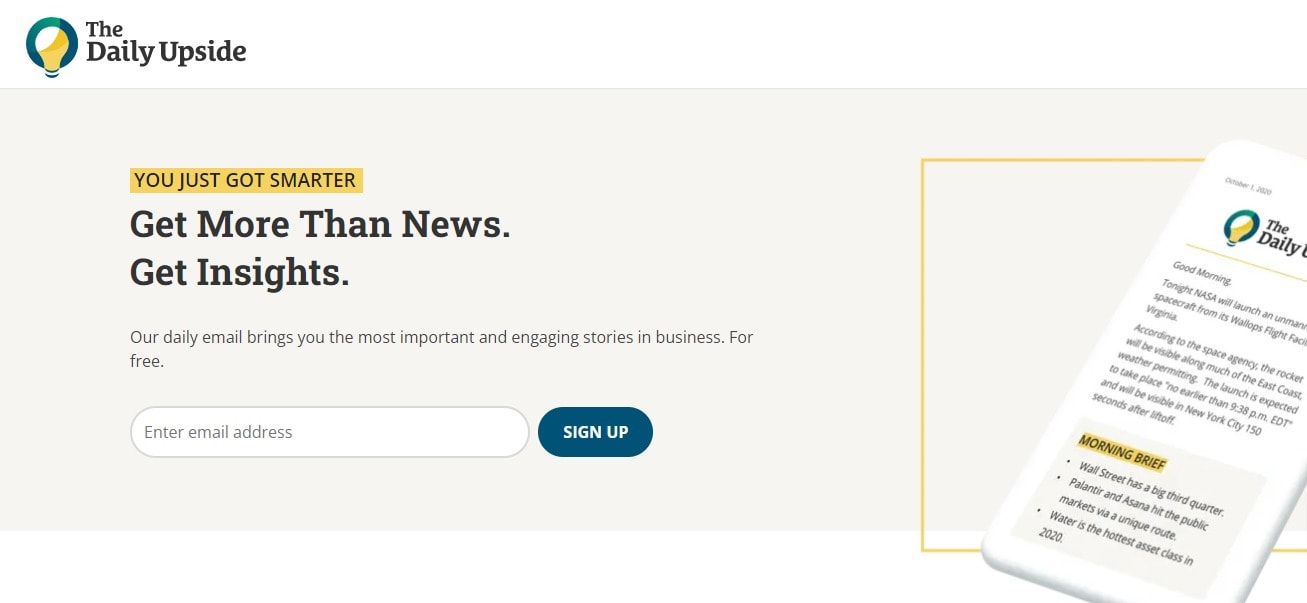The screenshot features an email subscription invitation from "The Daily Upside." In the upper left corner, the company name "Daily Upside" is displayed in dark gray font, with "The" in a much smaller font positioned above the "D" and to the left. Accompanying the text is the company logo: a half-white, half-gold light bulb enclosed within a greenish-gray circle.

The background of the image has a very light gray hue. On the left side, bold dark gray capital letters highlighted in a gold color state "YOU JUST GOT SMARTER." Below that, in larger font, it reads, "Get more than news, get insights." Continuing down, in regular font, the caption mentions, "Our daily email brings you the most important and engaging stories in business for free."

Further down, there's a white rectangular box with rounded corners instructing users to "Enter email address." To its right, a greenish-blue button labeled "Sign Up" in white font is displayed.

On the right side of the image, there's an illustration resembling a sheet of paper, showing a partial view of "The Daily Upside" logo. Below it, the text "Good Morning" appears, although the rest is not fully readable. Underneath this, a headline in capital letters highlighted in gold states "MORNING BRIEF," followed by, "Wall Street had a big third quarter," along with a few additional lines of text.